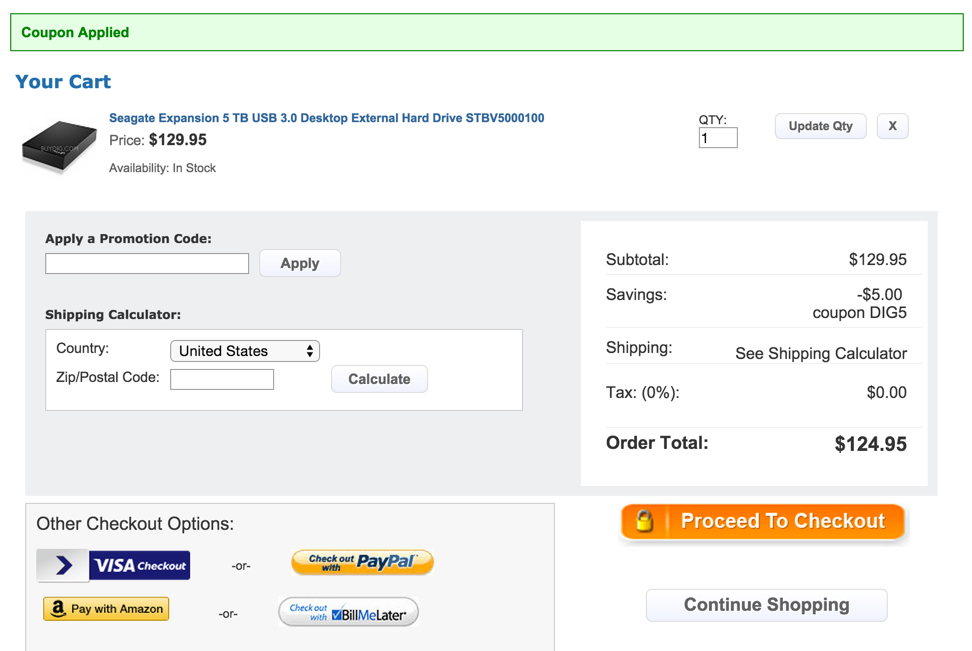This digital image presents a detailed view of an online shopping cart interface. At the top of the screen, there is a green bar indicating that a coupon has been applied. Below that, the heading "Your Cart" is prominently displayed.

The main section showcases a Seagate Expansion 5TB USB 3.0 Desktop External Hard Drive (Model: STBV5100) priced at $129.95, with a selected quantity of one unit. There is an "Update Quantity" button available for quantity adjustments. The item is listed as "In Stock."

Further down, users have the option to "Apply a Promotion Code." Below the itemized list, the subtotal is shown as $129.95, complemented by a "$5 Coupon Savings" deducted from the subtotal. Shipping costs are determined via a "Shipping Calculator," although no specific shipping fee is indicated. The tax rate is displayed as 0%, with the tax amount being $0.00, bringing the order total to $124.95.

At the bottom of the cart, users are presented with multiple action buttons. The prominent "Proceed to Checkout" button is orange and features a small lock icon, signifying a secure transaction. Additionally, there are "Continue Shopping," "Paypal," and "Fill Me Later" buttons, along with options for "Visa Checkout" and "Pay with Amazon."